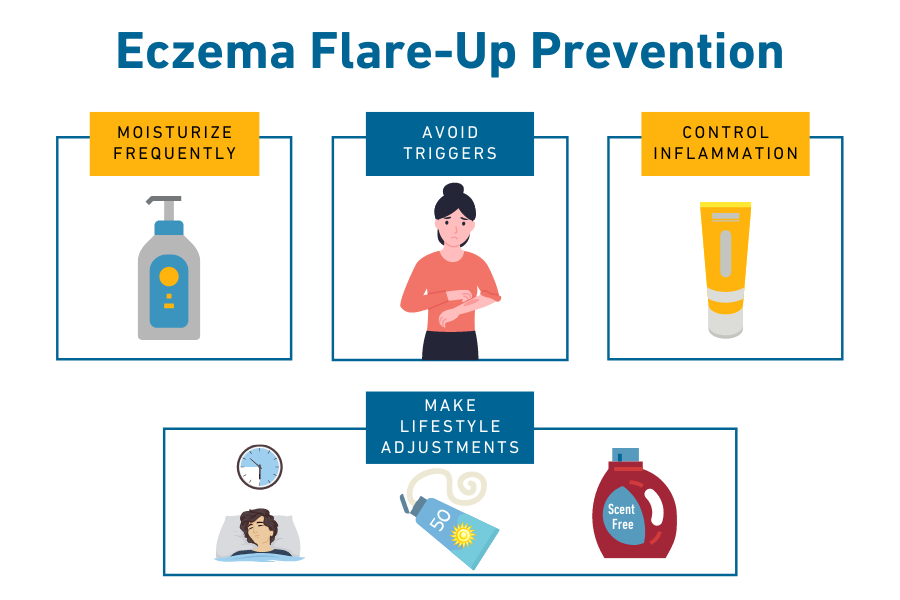This infographic, set against a white background, is designed to provide tips for eczema flare-up prevention. At the top, the title "Eczema Flare-Up Prevention" is prominently displayed. Below it, three squares are aligned horizontally, each containing an illustration with accompanying instructions.

- **First Square:**
  - *Top Rectangle:* A maroon-colored rectangle with orange text reading "Moisturize Frequently."
  - *Illustration:* A detailed pump bottle in shades of grey, blue, and yellow.

- **Second Square:**
  - *Top Rectangle:* A dark blue rectangle with white text that says "Avoid Triggers."
  - *Illustration:* A woman with black hair wearing a long-sleeve salmon-colored jersey and dark pants.

- **Third Square:**
  - *Top Rectangle:* An orange rectangle with text in maroon or dark blue, reading "Control Inflammation."
  - *Illustration:* A yellow tube with a white lid.

Below these squares, a larger landscape rectangle includes additional lifestyle tips:

- *Left Illustration:* A person sleeping with a clock above them, emphasizing the importance of sufficient sleep.
- *Middle Illustration:* A sunscreen bottle with some squeezed-out sunscreen next to it.
- *Right Illustration:* A red bottle of scent-free laundry detergent.

The blue rectangle above these illustrations advises to "Make Lifestyle Adjustments."